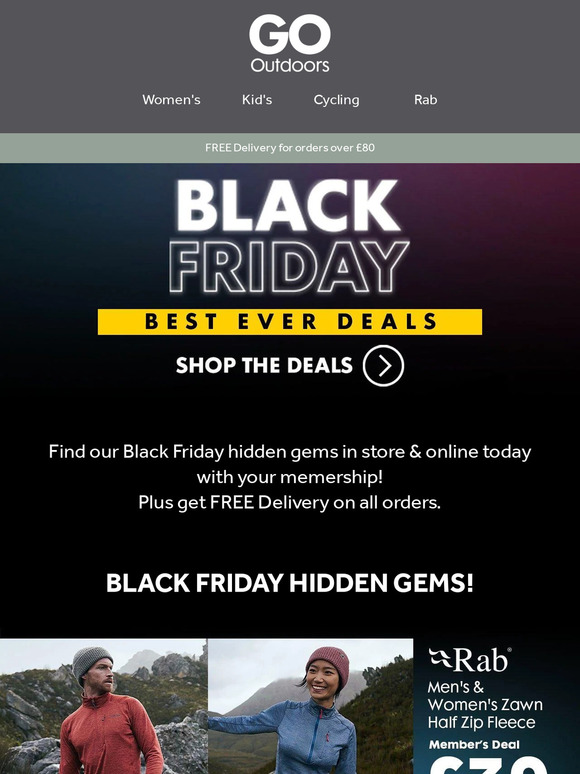This promotional image prominently features a banner promoting outdoor gear from a retailer. At the top, the text "Go Outdoors" is displayed, accompanied by various categories including Women's, Kids, Cycling, and Rab, emphasizing a broad range of products. A notable promotion includes "Free Delivery for Orders Over £80." The image highlights "Black Friday Best Ever Deals" with a visually striking "Shop Deals" button, featured prominently in a white circular icon.

Additionally, the ad encourages customers to discover Black Friday hidden gems both in-store and online through their membership, which also offers the perk of free delivery on all orders. Underneath, there's an image of a man and a woman modeling athletic wear; the man sports a red long-sleeve fitness shirt paired with a gray cap, while the woman wears a blue full-sleeve workout outfit with a red cap. This section promotes the "Rab Men's and Women's Zon Hap Zip Fleece," exclusively available for members.

The overall design features a contrasting color scheme with a dominant black background, accented by a gray top section with white text. A vibrant yellow section labeled "Best Ever Deals" adds a touch of brightness, drawing attention to the promotional content, characteristic of seasonal holiday sales.